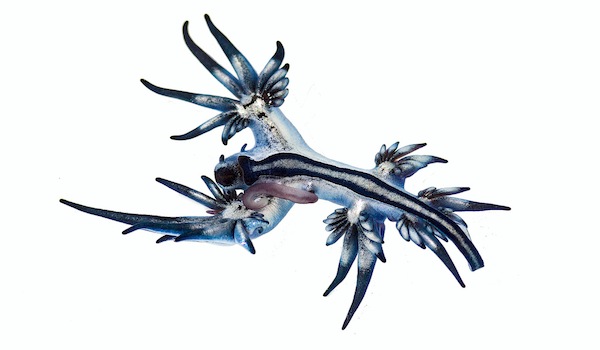This detailed drawing features an imaginative and fantastical blue sea creature with a light blue body set against a clear white background. The creature displays a variety of tentacle formations: two prominent front tentacles that split into smaller tentacles, a V-shaped tentacle extending from the bottom, and two tentacles at the rear resembling a tail. It possesses a stripe marked by two black lines with a white center that runs from the lower right to the upper left section of the body, giving the appearance of a Y-shape where two tentacle branches emerge upward, exhibiting black tips. A grey worm-like figure sits on one of the front tentacles, seemingly being consumed by the creature. The elaborately detailed tentacles are mainly black with blue hues, emphasizing its enigmatic and otherworldly design.